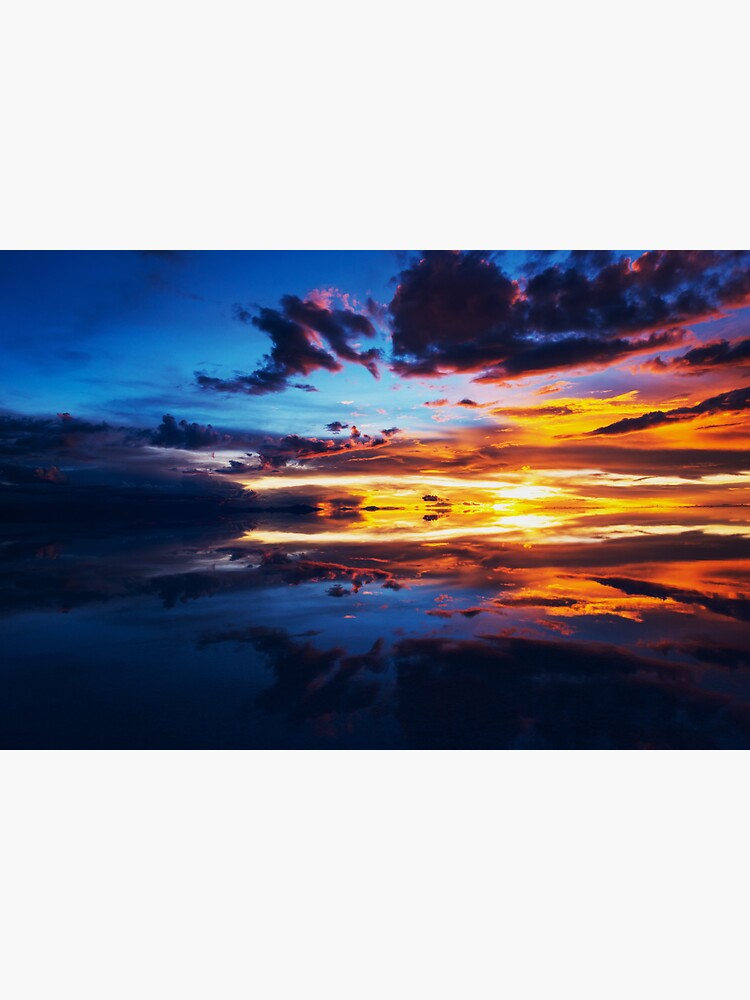In the photograph, an outdoor scene captures the mesmerizing moment of a sunset over an expansive body of water, possibly the ocean. The upper sky is a tapestry of deep blues, gradually giving way to dark clouds streaked with vibrant amber hues from the setting sun. This amber coloring seamlessly spills onto the water below, creating a breathtaking reflection that lends a three-dimensional quality to the image. The waterfront is so shrouded in shadows that it's challenging to distinguish where the land ends and the water begins, adding a sense of mystery to the scene. Rich in colors ranging from bright yellows, oranges, and reds to touches of pinks, purples, and even hints of green, the sky and water blend into a stunning visual symphony. The absence of human figures allows the viewer to fully immerse in the beauty and tranquility of this captivating sunset.